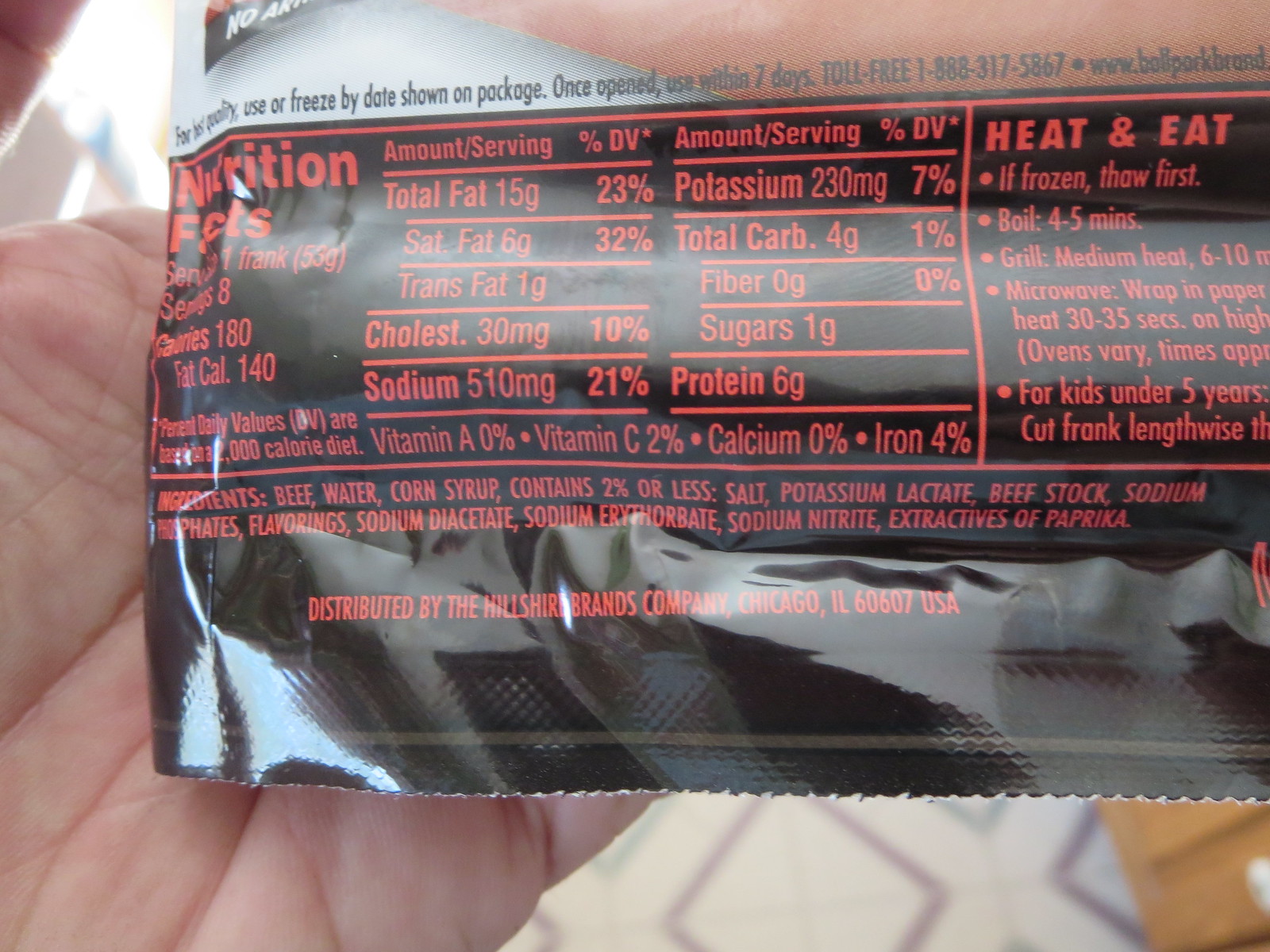In this realistic photograph, a person’s hand is prominently featured as it grasps a package. The hand, positioned on the left side of the image, reveals a wrinkled palm and part of the thumb in the top left corner. Beneath the hand, the floor is visible and characterized by square patterns. The object being held appears to be a product wrapper.

At the top of the wrapper, there is a partially obscured image. The central section is black with nutritional information displayed prominently in red text. The details of the nutrition facts include the following: total fat 15 grams, saturated fat 6 grams, trans fat 1 gram, cholesterol 30 milligrams, sodium 510 milligrams, potassium 230 milligrams, total carbohydrates 4 grams, fiber 0 grams, sugar 1 gram, and protein 6 grams.

On the right side of the wrapper, there are instructions for cooking. It advises to "heat and eat," with the following specific directions: "If frozen, thaw first. Boil for 4 to 5 minutes. Grill over medium heat for 6 to 10 minutes. Microwave by wrapping in paper and heating for 30 seconds."